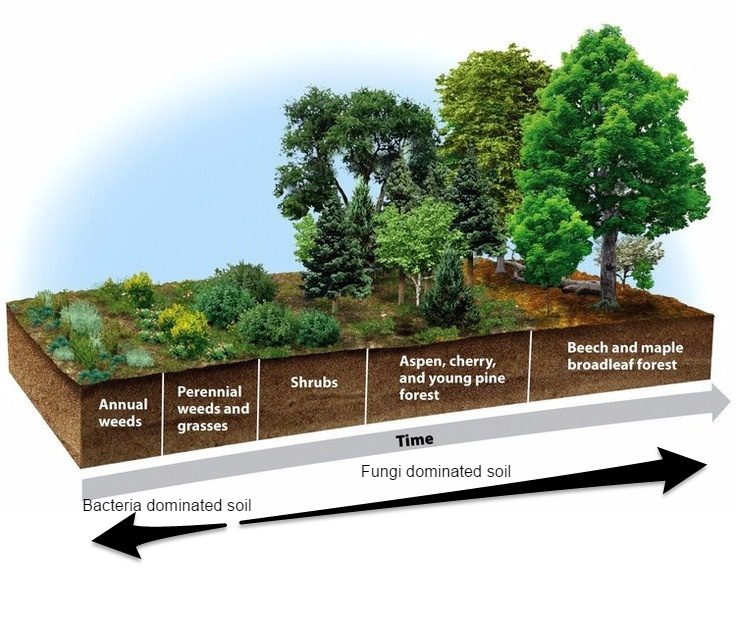The image is a detailed scientific diagram, combining elements of illustration to depict plant succession over time. The central feature is a raised rectangular 3D block of soil, illustrating the cross-section of earth with various plant types growing above it. The background features a blue sky, enhancing the pictorial representation.

The illustration is segmented into labeled sections from left to right. Beginning on the far left, the first label "annual weeds" shows a depiction of weeds typical for an annual growth cycle. Adjacent to this, "perennial weeds and grasses" indicate a variety of more persistent weeds and grasses. The next section, "shrubs," is represented by several green bushes. Progressing rightward, "aspen, cherry, and young pine forest" is illustrated with multiple young trees of these species growing closely together. Finally, "beech and maple broadleaf forest" is depicted featuring large, mature broadleaf trees.

Below the vegetation imagery, a prominent gray arrow spans the width of the diagram, pointing right and labeled "time" in its center, indicating the progression from left to right. Beneath this arrow, two smaller black arrows point in opposite directions. The arrow pointing left is labeled "bacterial-dominated soil," aligning with the sections depicting weeds, whereas the right-pointing arrow is labeled "fungi-dominated soil," aligning with the mature tree stages.

This detailed diagram comprehensively illustrates the natural progression of plant growth and soil changes over time, from bacterial dominance associated with early plant stages to fungal dominance in mature forest ecosystems.